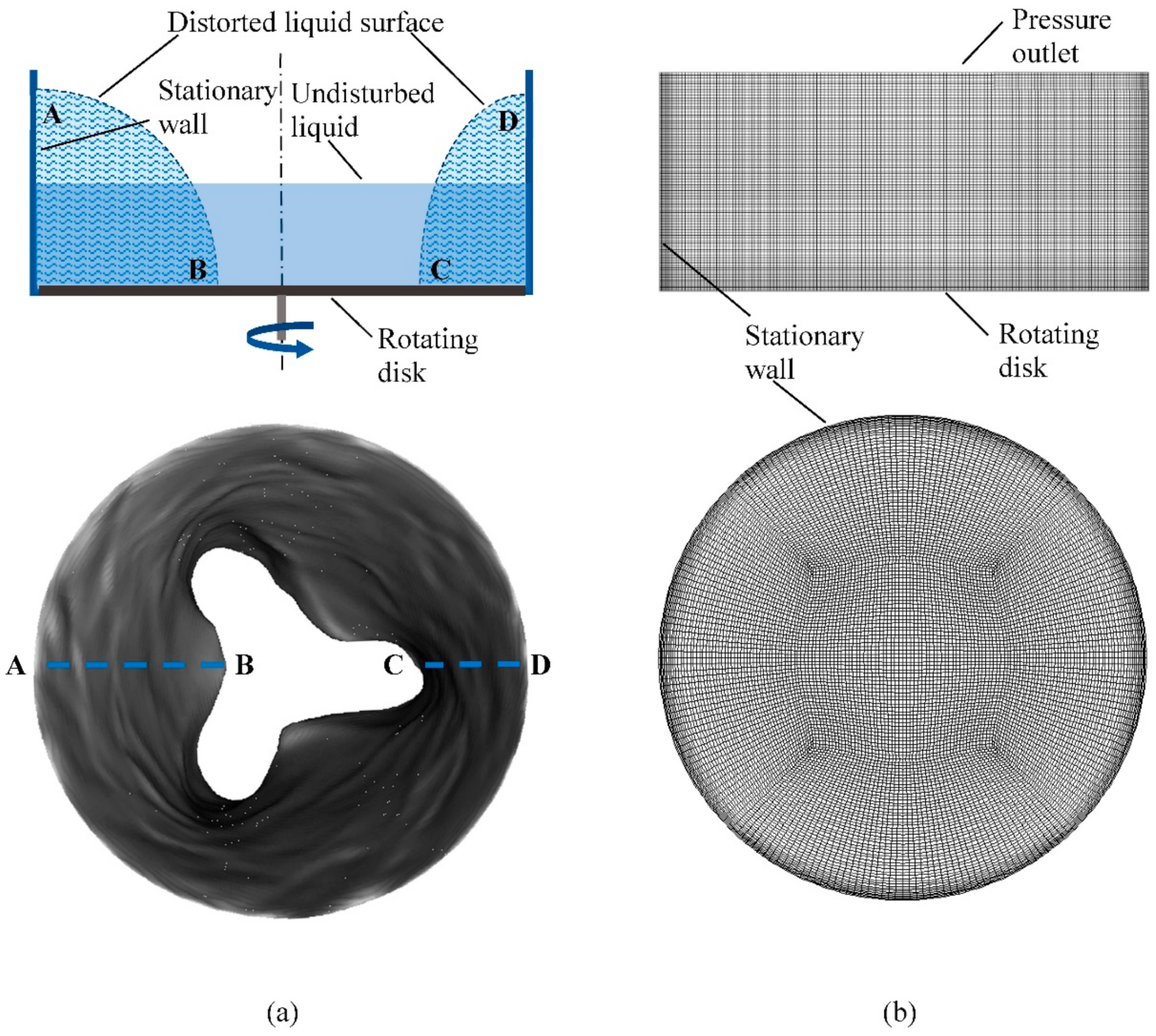This scientific diagram consists of two primary sections, each with a distinct layout and labeling. The left section is labeled "distorted liquid surface" and is divided into two parts. The left part features a schematic showing a "stationary wall" and contains labeled segments "A" and "B." The right part shows "undisturbed liquid" with segments "C" and "D." Below this section, there is a black circle marked with the letters "A, B, C, D," and further below, "A" is indicated in parentheses.

The right section of the diagram is predominantly in black and white, featuring a plaid design. At the top, it is labeled "pressure outlet," beneath which is "stationary wall" and "rotating disk." This schematic is visually distinct due to its plaid pattern. Below this section, another circle with a similar plaid pattern is labeled with "B" in parentheses.

Both sections include diagrams illustrating interactions at and below the waterline, capturing varying surfaces, pressures, and structures.